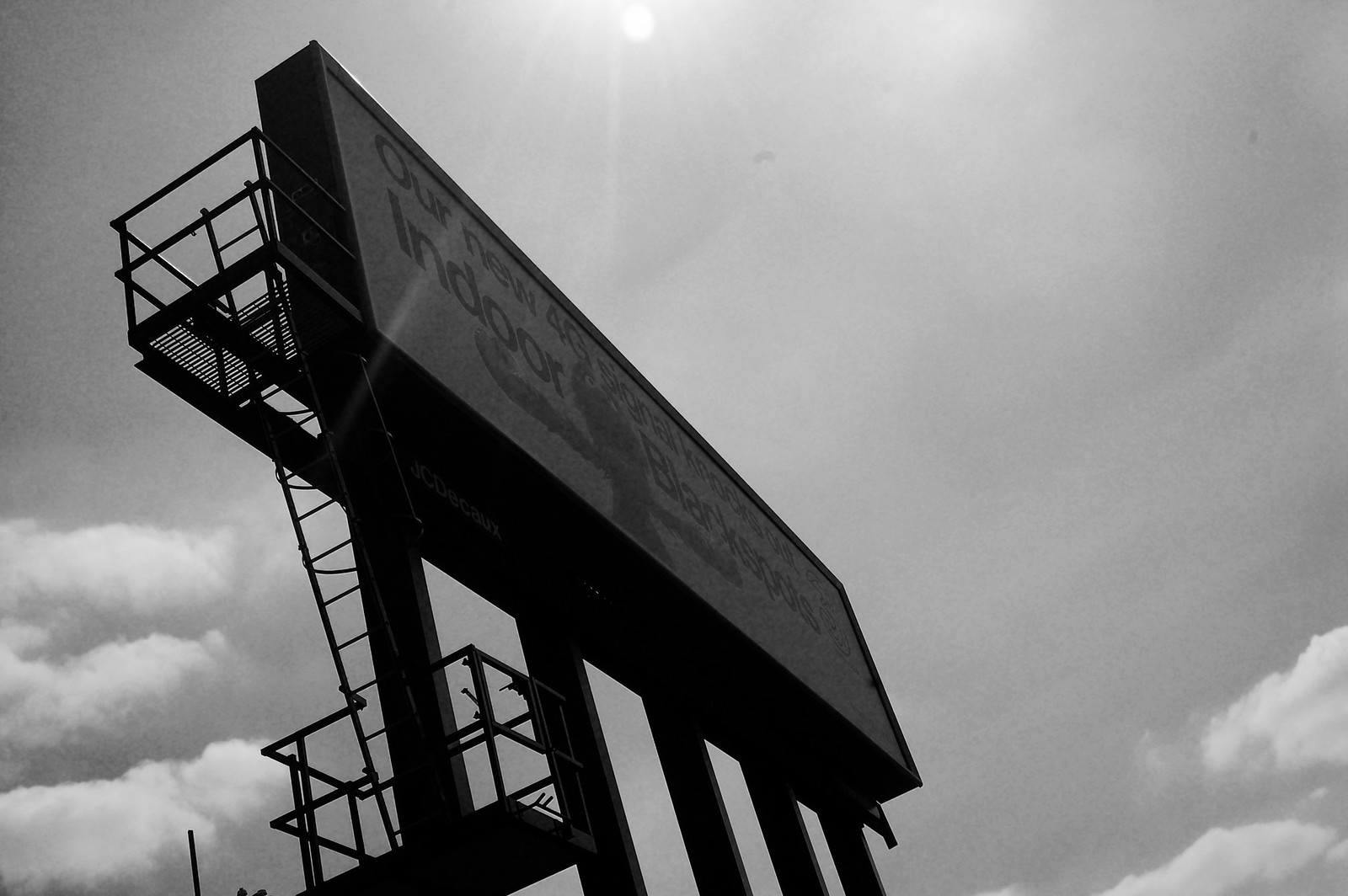The black and white photograph is taken from a low, upward-pointing angle, presenting a dramatic view of a giant billboard supported by five large steel beams. The camera angle is from the perspective of someone looking up at the sky, capturing the lower, underside of the billboard structure as well as its front. The sun's glare is visible at the top middle of the image, with streaks of sunlight adding contrast to the scene. Fluffy white clouds populate the sky, concentrated in the bottom right and left corners. The billboard's text is partially legible, displaying the words "Our New" followed by "Indoor" amidst the otherwise unreadable writing. A ladder and catwalk can be seen attached to the back of the billboard, indicating access for maintenance or ad changes.